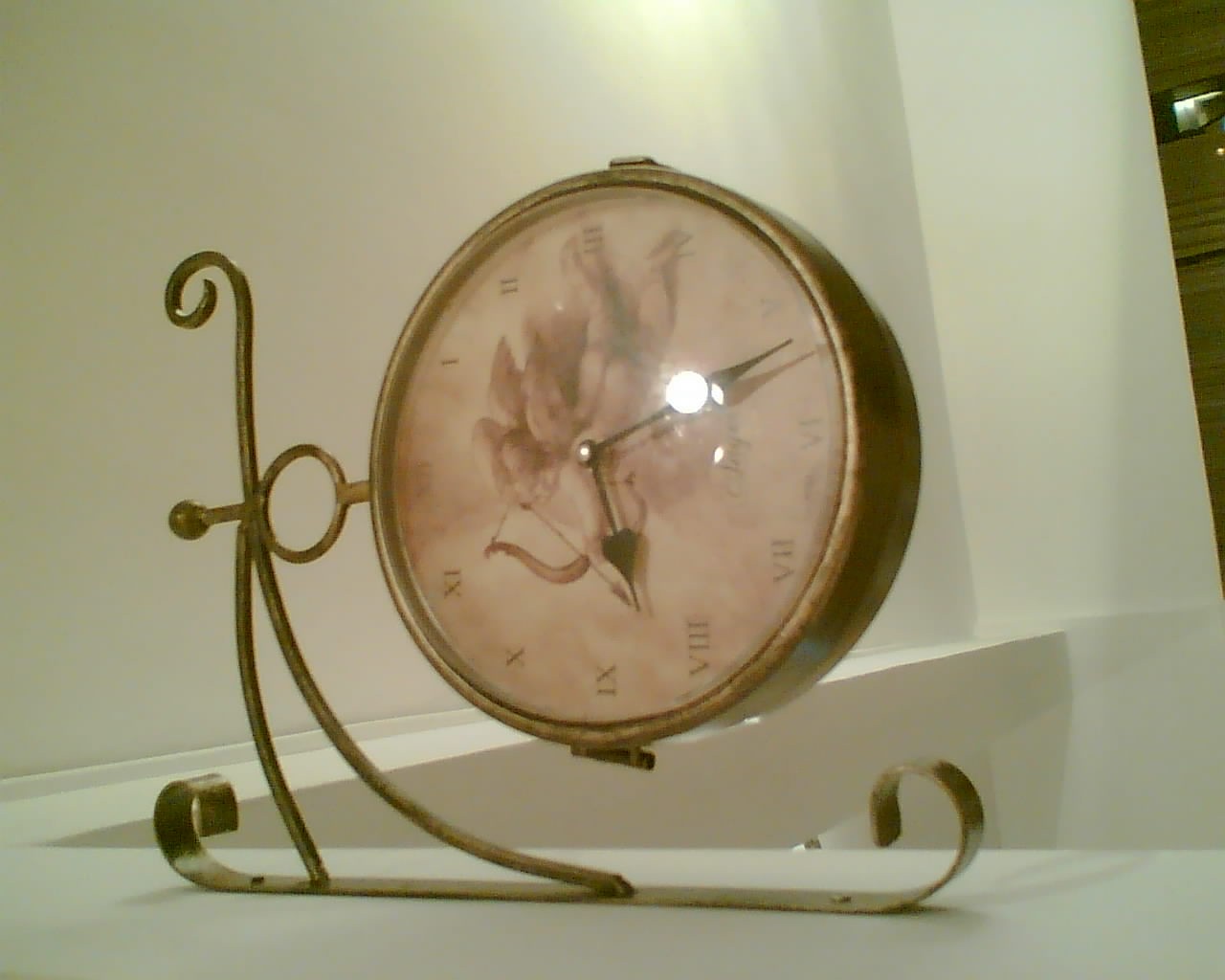This image showcases a brass clock set against a stark white background comprising various white shapes that resemble walls or a ceiling. The brass clock features an intricate design with a flat body that curls up at the ends, forming two long, triangular pieces with a circular slope instead of a flat line. These pieces converge into a point adorned with a small curl. A circular ornament adjacent to these elements is attached to the clock's main body, which is a large circle bordered with golden brass. The interior of the clock boasts an antique peach-brown face adorned with nearly cloud-like oval shapes, further enhancing its vintage allure. A noticeable glare covers the clock's face, partially obscuring the black hands, adding a touch of elegance and reflecting light in a way that highlights its aged beauty.